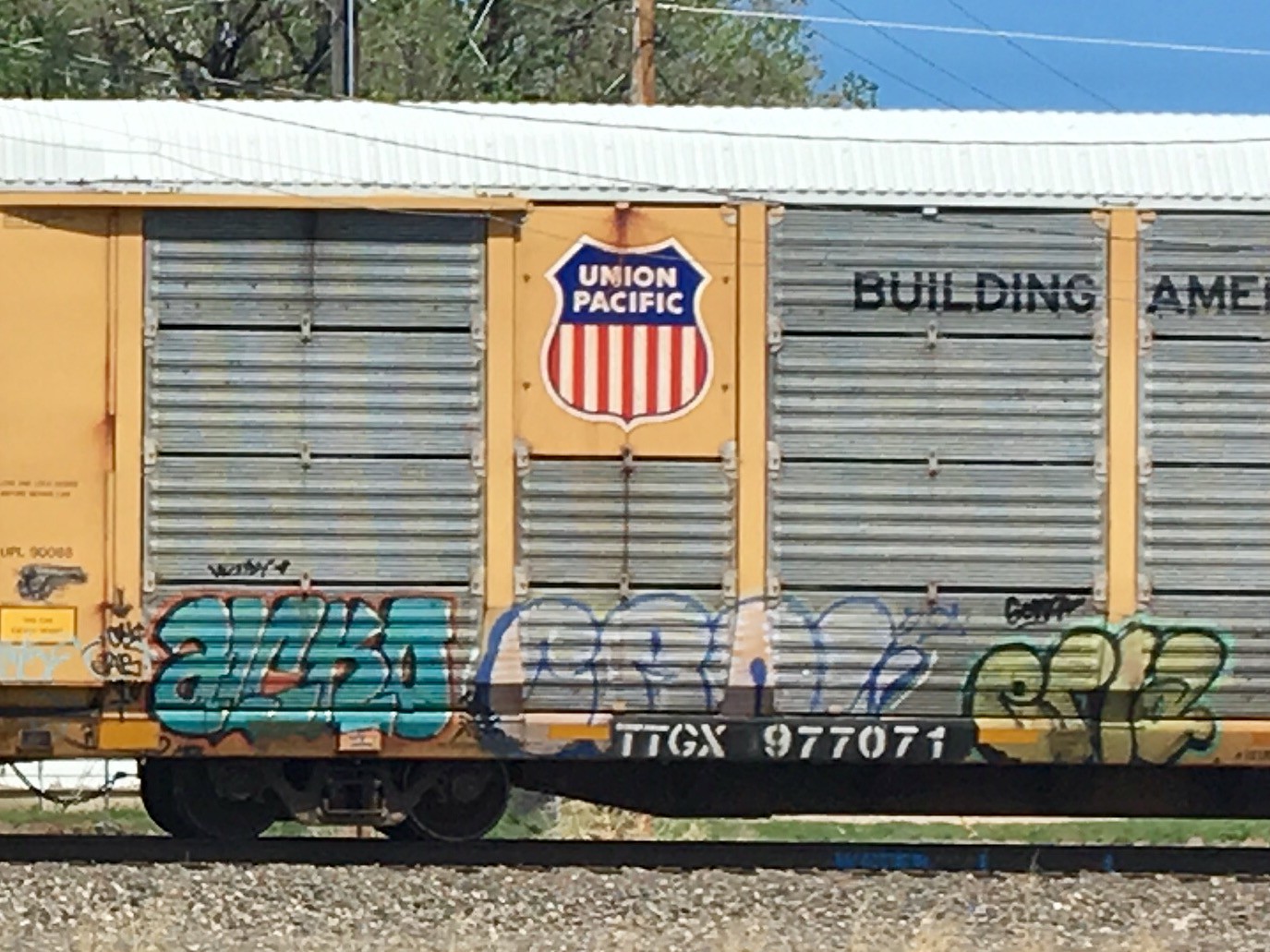The image features a detailed close-up of a Union Pacific train car, partially cut off at the edges. The train car sits on black tracks with slight blue graffiti, surrounded by light gray gravel. The yellow train car has a combination of orange sides and a white roof, with metallic gray doors along its length. The bottom of the car is adorned with multicolored graffiti in blue, gray, and yellow hues. The Union Pacific logo, a red-and-white striped shield with a blue top, is prominently displayed in the center. Above the logo, “BUILDING AMERICA” is written in black text. The car bears the identification number TTGX 977071 in white letters at the bottom right. In the background, a power line stretches over the train, with a large green tree and a clear blue sky enhancing the scene.